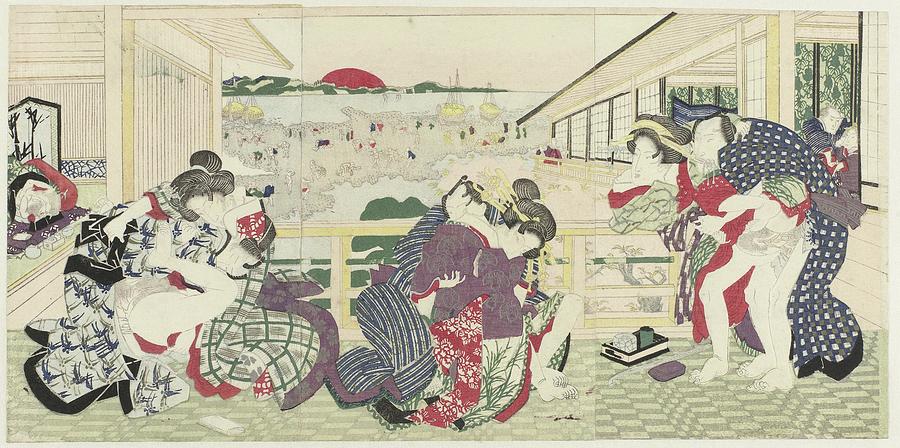The illustration depicts a traditional Japanese scene with various couples and individuals depicted in distinct poses. The artwork prominently features men dressed in long robes and women in vibrant kimonos, with their dark hair elegantly styled up and adorned with wooden hair sticks. The colors of their garments range from red to grey and purple, with some green patterns adding intricate details. The background showcases traditional Japanese architecture, including wooden structures and checkered windows. A striking red sun and lush green trees enhance the serene landscape, with additional buildings visible in the distance. The figures are positioned on a ground that appears to be covered by a green and beige rug, and the entire scene is set against an ivory-colored background. Furthermore, there are explicit depictions of intimate moments portrayed with remarkable clarity, wherein couples are engaged in various sexual positions, adding a distinct and provocative element to the overall composition. The art style is distinctly Japanese, characterized by its traditional aesthetic and evocative imagery.